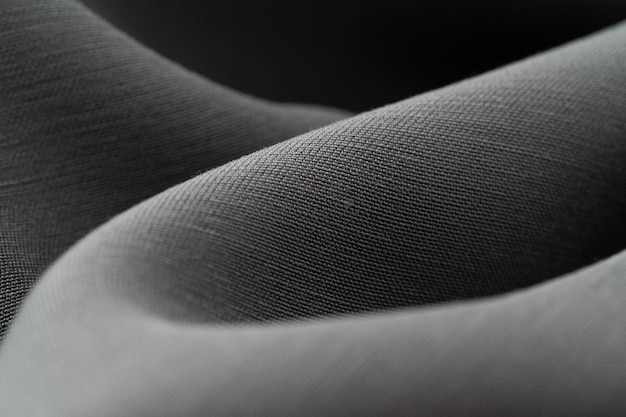This image is an intricate black-and-white digital photograph showcasing a detailed close-up of finely woven fabric. The fabric, predominantly in shades of gray and black, features a grid or crisscross knit pattern, suggesting a cotton-like texture. The photograph highlights the delicate stitching and intricate weave, making the material's folds and contours highly visible. The fabric in the foreground wraps from the upper right to the lower left and back around, while another part of the same fabric appears in the background on the left. Both pieces appear to be the same material. A black background surrounds the fabric, creating a stark contrast that emphasizes the fabric's details. The image is slightly blurred at the front and back left, adding depth and dimension to the photograph.